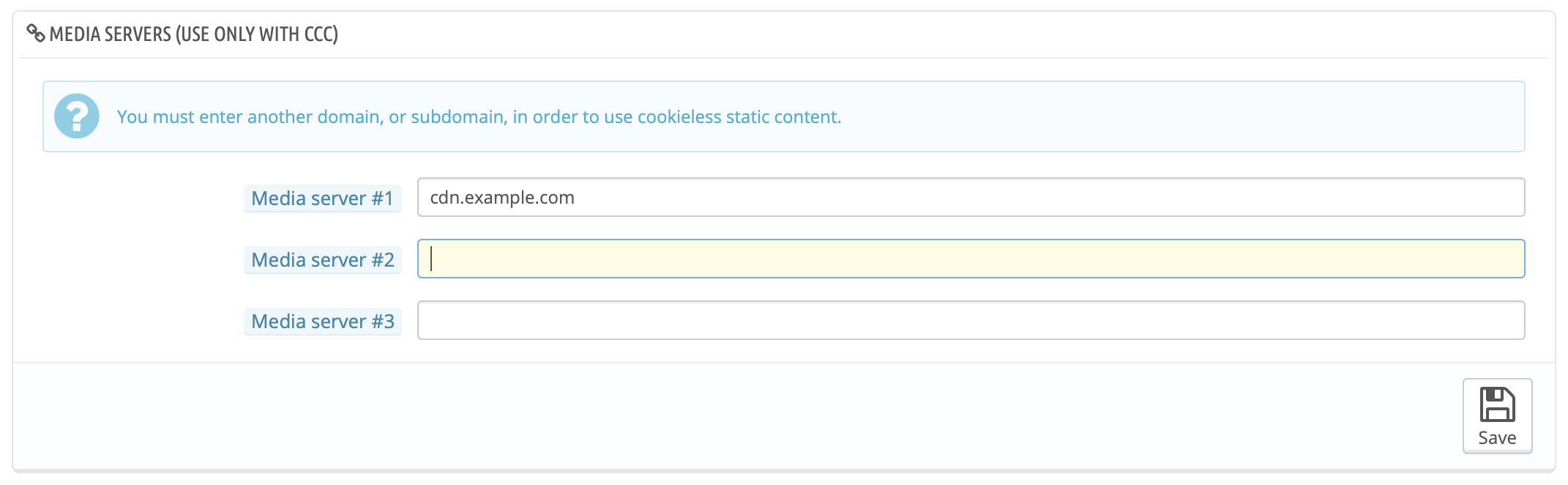Caption:
The image displays a settings interface for managing media servers. In the top left corner, there is black text that reads, "Media Servers (Use Only with CCC)." Below it, blue text prompts, "You must enter another domain or subdomain in order to use the cookie list."

The detailed settings are as follows:
1. Media Server Number One: cdn.example.com
2. Media Server Number Two: [Input field]
3. Media Server Number Three: [Red square input field]

In the bottom right corner, a floppy disk icon indicates a save option. The background consists of various elements, representing different features and functionalities associated with configuring media servers.